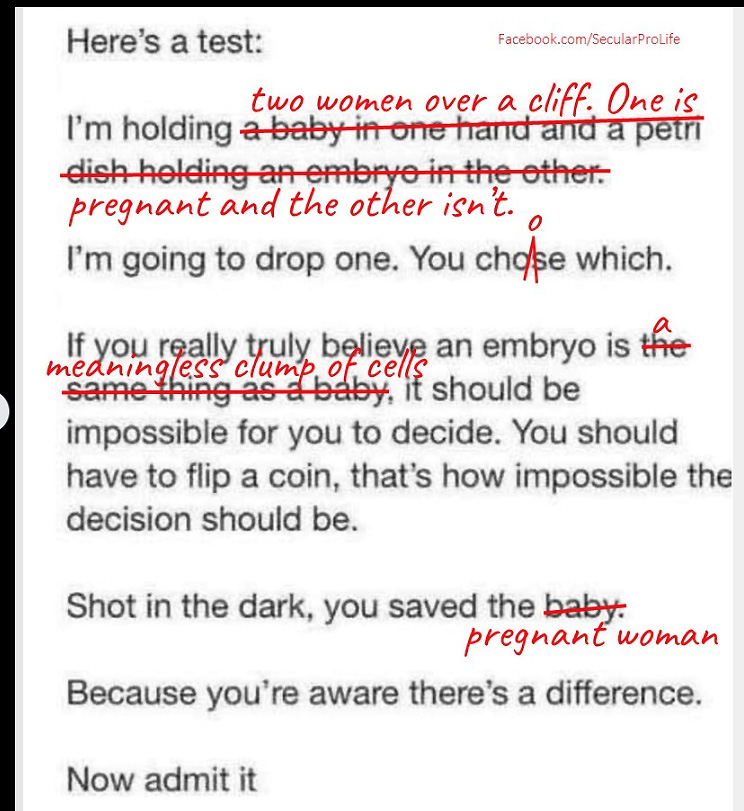In the image, there is a thin black bar running vertically on the left side and extending horizontally from the upper left to the upper right. At the top, in black text, is the phrase "Here's a test." Positioned on the right-hand side, in much smaller print, is the URL "facebook.com/secularprolife."

The main content of the image features red and black text alterations over an original message. Initially, the text stated, "I’m holding a baby in one hand and a petri dish containing an embryo in the other," but "baby in one hand and a petri dish containing the embryo in the other" is scratched out in red. It has been replaced to depict "two women over a cliff, one is pregnant the other isn’t."

Following this change, the black text continues: "I’m going to drop one. You choose." Here, "choose" is initially misspelled with an additional 'O,' which is corrected in red ink. The next line reads: "If you truly believe an embryo is," with the phrase "the same thing as a baby" scratched out in red and replaced with "a meaningless clump of cells."

The following line asserts, "It should be possible to flip a coin before you decide. How is it possible the decision should be made..." The original sentence likely ended differently but is interrupted by the alteration, continuing with "shot in the dark you save the baby," where "baby" is once again scratched out and replaced in red with "a pregnant woman."

The image concludes with the red-inked phrase: "because you’re now aware there's a difference. Now admit it." This acts as a closing statement addressing the viewer with a challenge to their beliefs outlined in the altered text.